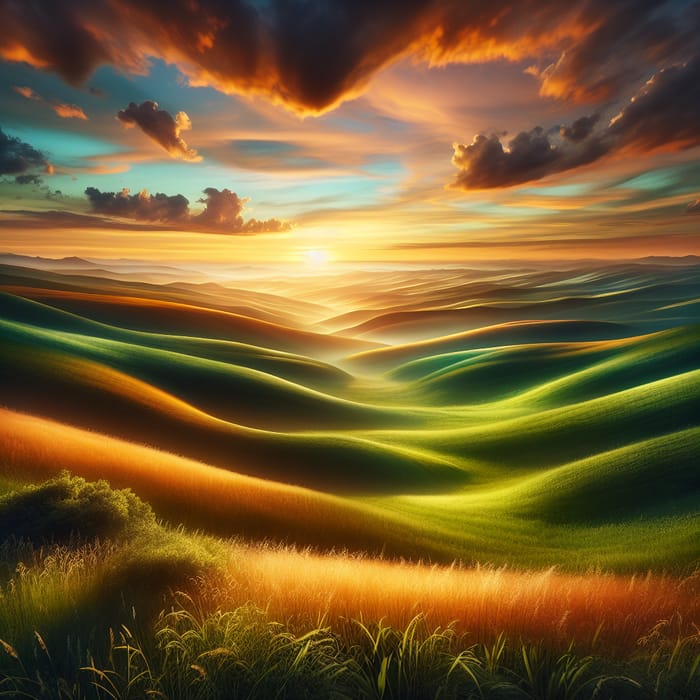An AI-generated outdoor scene depicting an abstract and surreal landscape. The dark blue sky transitions into hues of orange, with sunshine piercing through scattered, realistic-looking clouds. The foreground features patches of green grass interspersed with golden, hay-like weeds. Rolling, hyper-stylized hills in varied shades of green, brown, and teal create a wave-like appearance, almost resembling an ocean. Some artifacting is visible at the bottom, where a field of wheat blends into leafy textures. A distant building or house can barely be discerned, shrouded in fog and the fading light of either a setting or rising sun, projecting a soft glow across the undulating terrain.